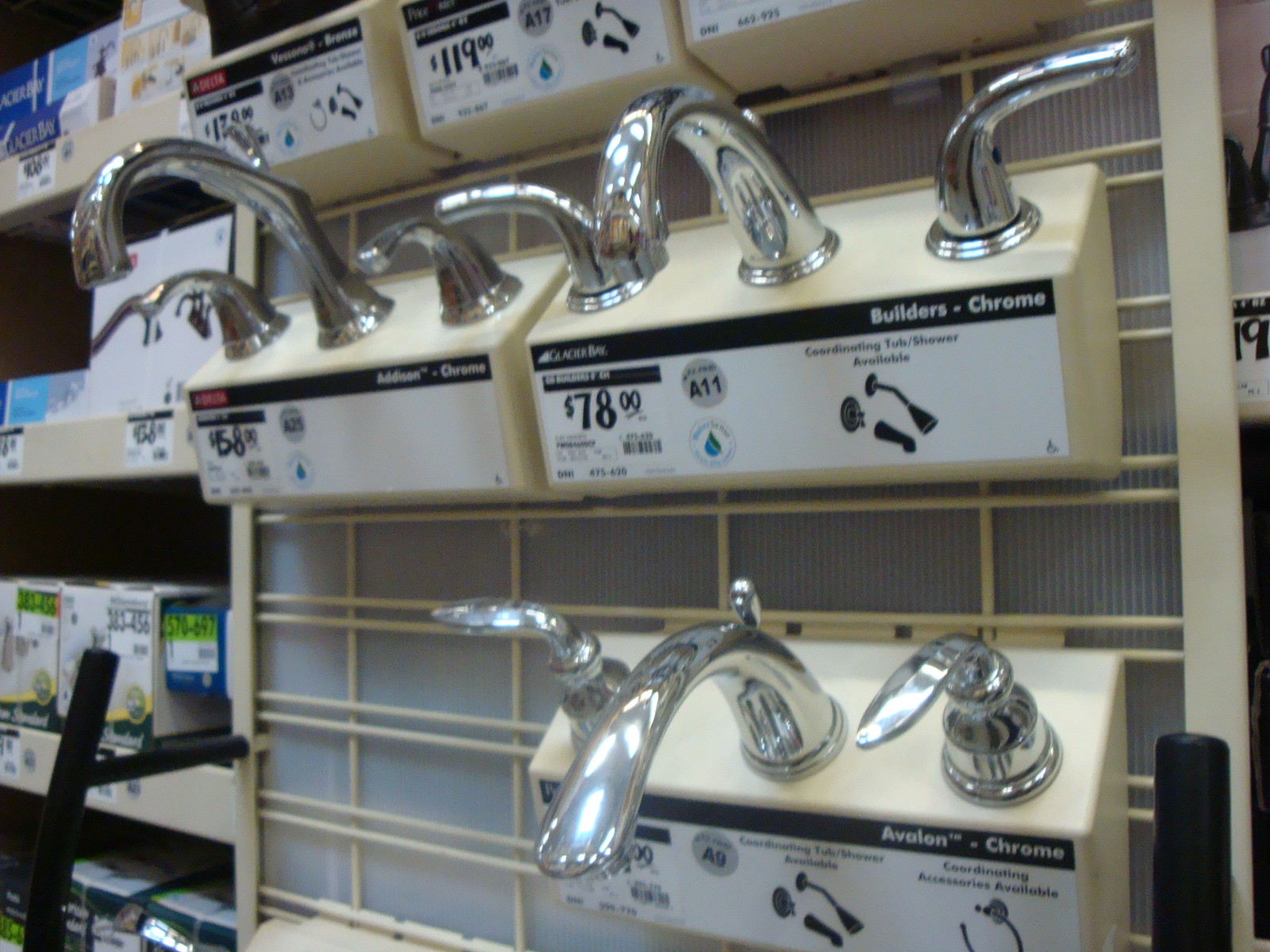This color photograph showcases a detailed display of sink and kitchen faucets in a hardware store. The display is mounted on an ivory metal structure with grating, set against a white ridged backdrop. There are three featured chrome faucets, each with a polished finish. The faucets have a central spout flanked by hot and cold water knobs. The top left faucet, labeled Edison Chrome, stands taller and is priced at $158.99. To its right, the Builders Chrome faucet, featuring a simple curve, is marked at $78. The bottom right faucet, Avalon Chrome, extends further out with a soft curve, though its price is obscured. Each faucet is accompanied by a white and black information label detailing the product name and price. To the left of the display, blurred tan-colored shelves with boxed products are visible, suggesting additional hardware items, though their specifics are indistinguishable.